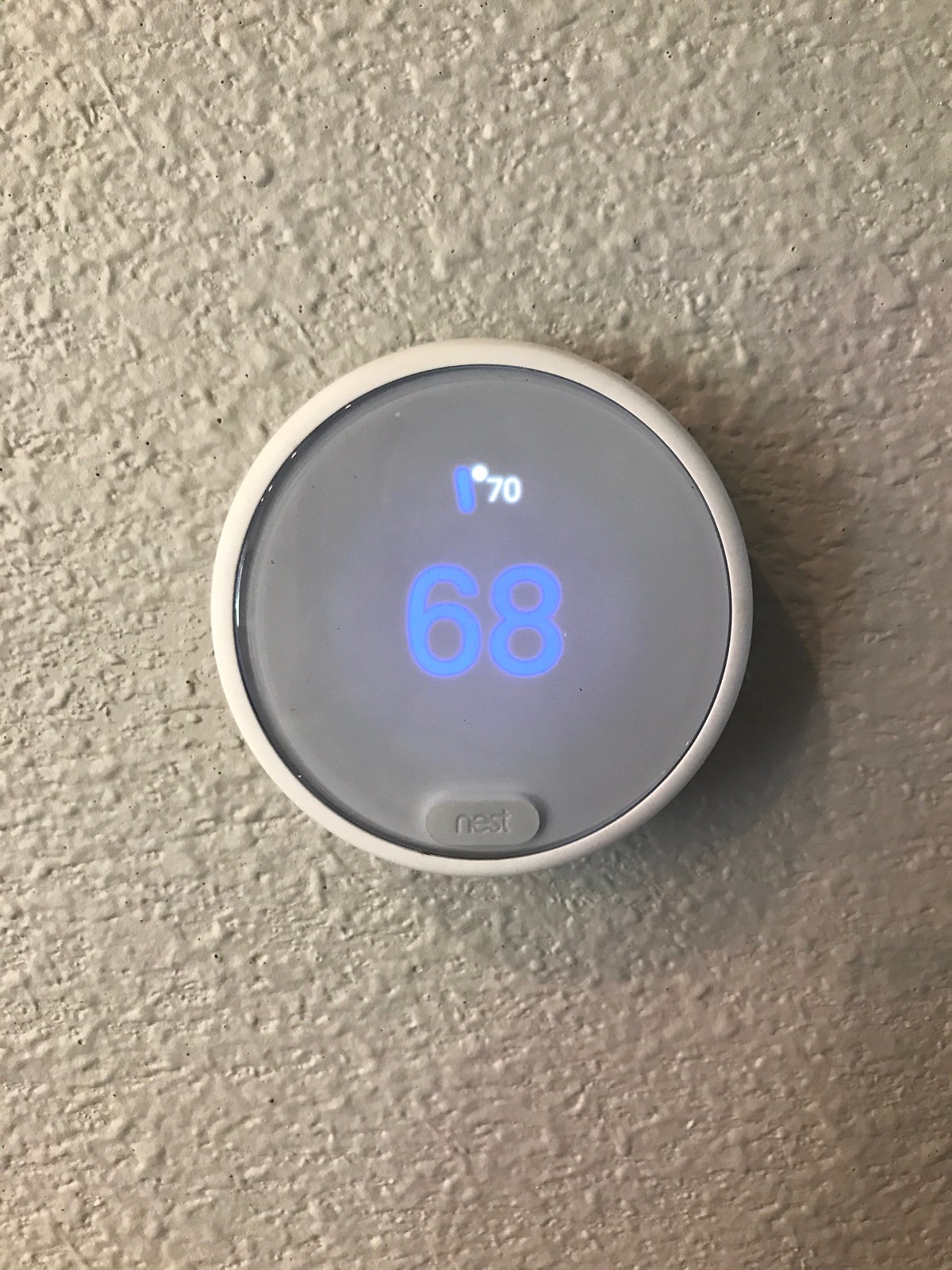The image showcases a wall-mounted Nest thermostat prominently displayed at the center. The wall, painted in an off-white cream color, features a noticeable bumpy texture with numerous small bumps and ridges, giving it a distinctly unsmooth appearance. The Nest device itself is characterized by a white circular rim encasing a gray screen. On this screen, the number "70" is displayed in white text, indicating the current setting. The design implies that the outer rim can be rotated to adjust the temperature, as suggested by a small line resembling an arrow. Additionally, the number "68" is presented in large blue text, likely representing the current room temperature. At the bottom of the screen, there is an engraved rectangular symbol with rounded edges, bearing the brand name "Nest" in all lowercase letters.